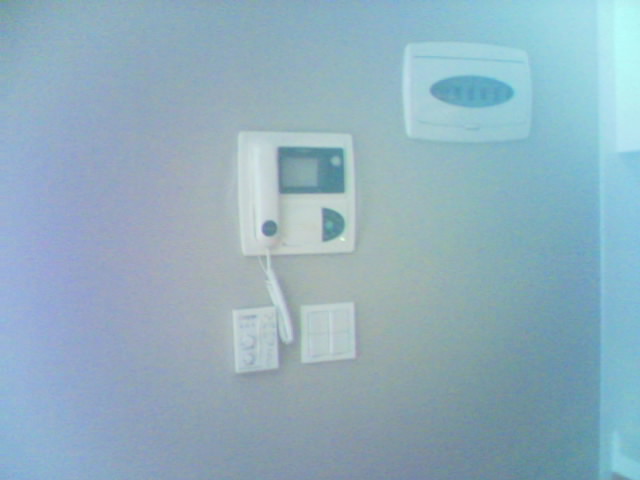The image showcases an off-white colored wall with subtle visual elements scattered across its surface. On the left side of the wall, there is a noticeable discoloration with patches of blue and hints of purple randomly appearing. Moving towards the center, there's a series of squares: a white square encloses a black square, which further encapsulates a smaller square that resembles a screen, though it is currently blank.

To the left of these squares is a telephone with a distinctive black dot on the receiver, and a white telephone cord extending down about two inches, touching another white outlet on the wall. Adjacent to this outlet is another white square that looks like a covered outlet of some kind.

In the upper right corner, there is a long white rectangle, approximately three inches in length, featuring a gray oval with faintly visible blue text inside. On the far right edge of the wall, the off-white surface meets a white edge, accompanied by a bit more of the purplish-blue shade seeping through.